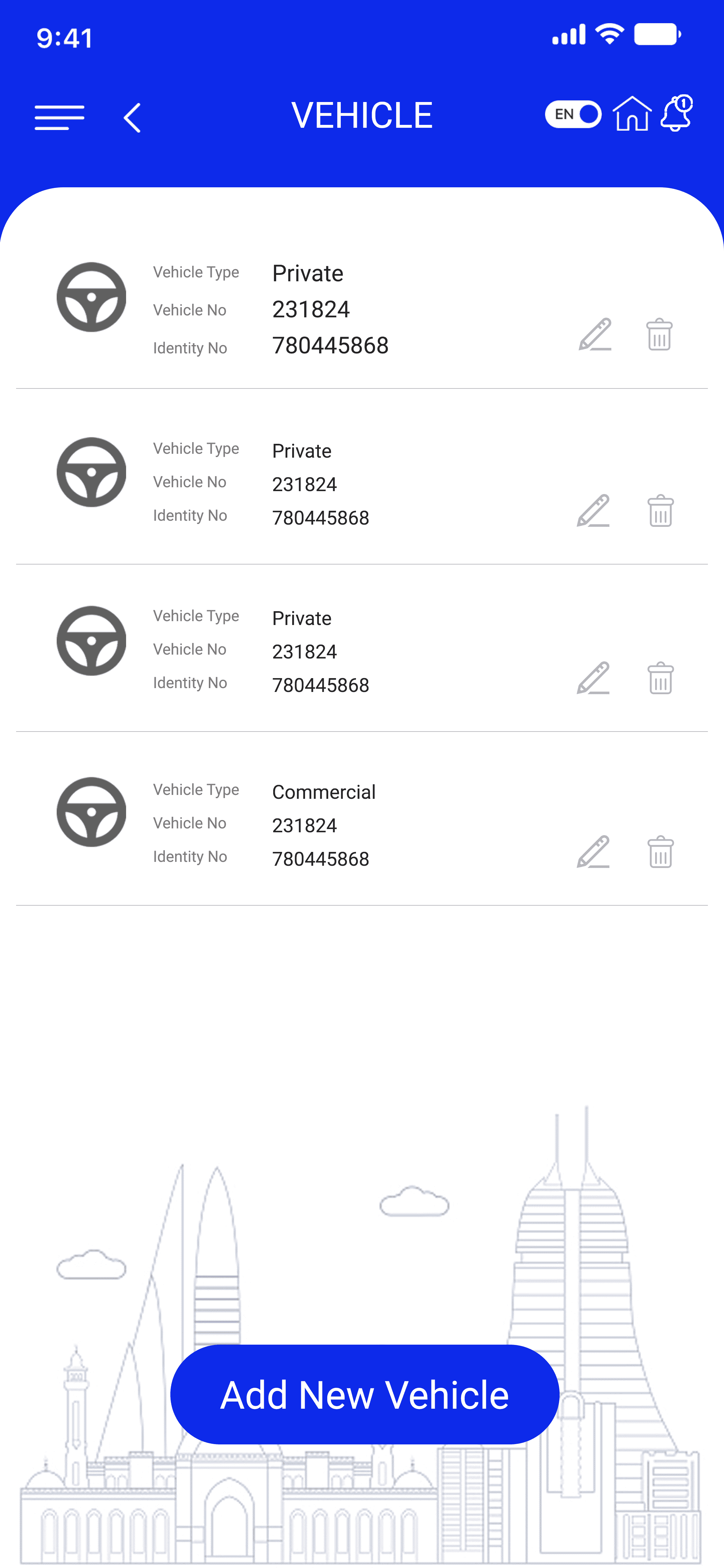This is a detailed screenshot from a smartphone screen displaying a vehicle management application interface. At the very top, a blue banner houses the time "9:41" in white on the left, along with a battery icon, network signal, and Wi-Fi indicator on the right. Below the banner, there's a navigation row featuring three horizontal lines, a back arrow (<), and the word "Vehicle" in white text. 

The main section starts with an icon for language selection labeled "EN" and a blue circle, followed by a home icon and a bell icon with a notification badge displaying the number one. Beneath this, various listed vehicles are shown, each accompanied by a steering wheel icon.

1. **Vehicle 1**
   - Vehicle Type: Private
   - Vehicle Number: 231824
   - Identity Number: 780445868
   - Edit Icon
   - Trash Can Icon

A thin gray divider line separates the entries.

2. **Vehicle 2**
   - Vehicle Type: Private
   - Vehicle Number: 231824
   - Identity Number: 780445868
   - Edit Icon
   - Trash Can Icon

3. **Vehicle 3**
   - Vehicle Type: Private
   - Vehicle Number: 231824
   - Identity Number: 780445868
   - Edit Icon
   - Trash Can Icon

4. **Vehicle 4**
   - Vehicle Type: Commercial
   - Vehicle Number: 231824
   - Identity Number: 780445868
   - Edit Icon
   - Trash Can Icon

At the bottom of the screen, there's a lightly drawn illustration in gray of a building with two clouds depicted in the sky. Centered below this artwork, a blue call-to-action button with white text stands out, prompting users to "Add New Vehicle."